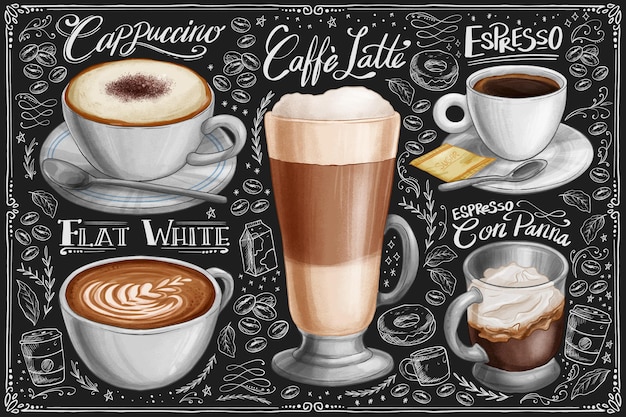The image is a detailed, artistic poster depicting various types of coffee on a black background, reminiscent of a coffee shop menu. The background is adorned with intricate white sketches of coffee-related items like milk jugs, coffee beans, donuts, and cups, adding a playful and elaborate touch. 

On the left top, there's a white cup and saucer with a cappuccino and a spoon beside it, accompanied by the text, "A cup of coffee and white oat bread." Below it is a white cup of flat white coffee featuring a delicate flower pattern on its surface. 

In the center of the poster, there's a tall, layered mug of café latte, clearly labeled "café latte" at the top. 

To the right, near the top, another white cup and saucer with an espresso and a yellow sugar packet is positioned. At the bottom right corner, there's a white mug filled with espresso con panna, topped with a swirl of whipped cream, creating a rich and creamy presentation. 

Each coffee variety is named in distinct white fonts, enhancing the visual appeal and clearly identifying the different types of coffee. The entire backdrop is filled with whimsical white sketches of coffee beans, donuts, milk cans, leaves, and cups, making the poster lively and visually engaging.